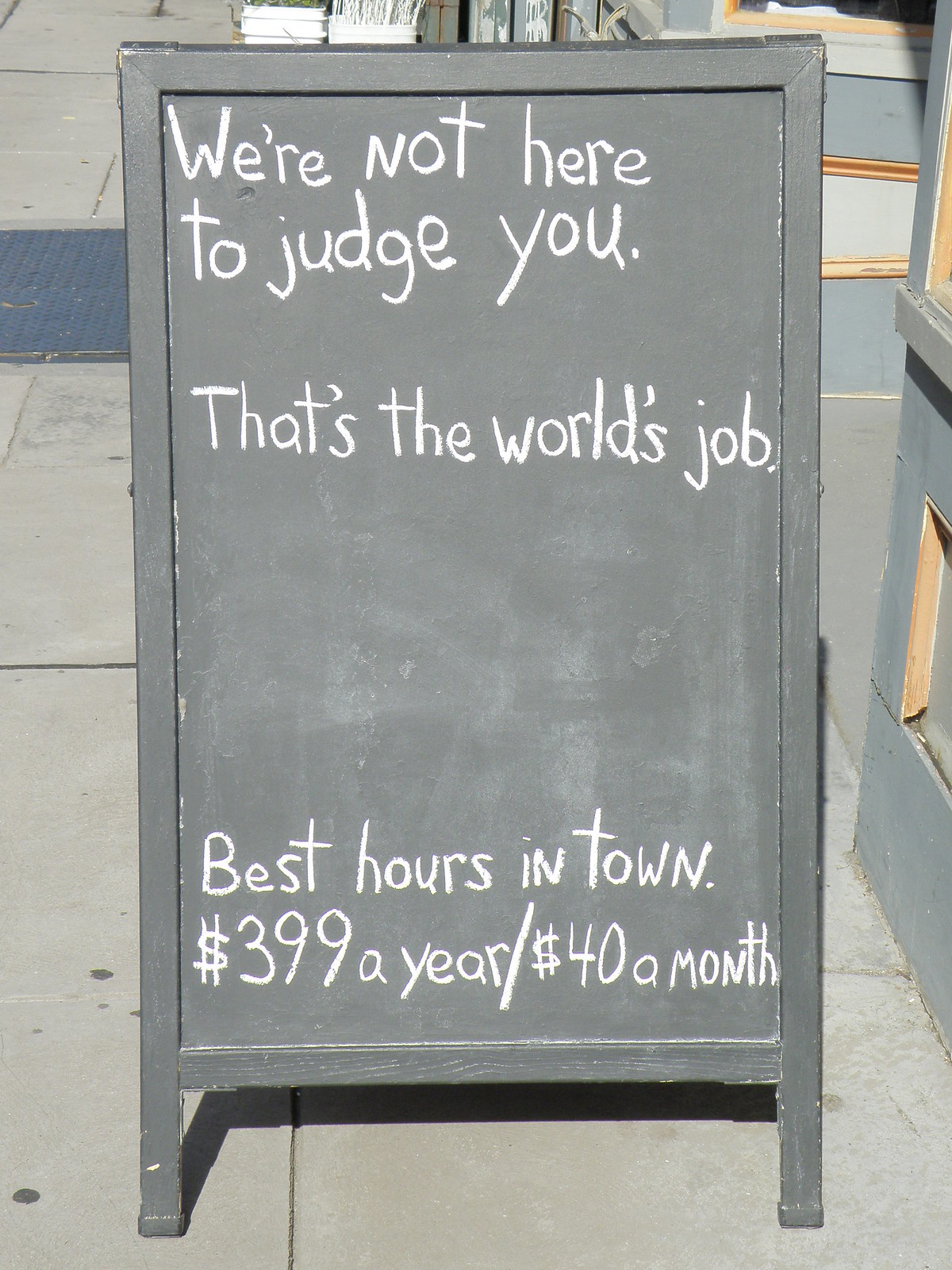This detailed image depicts a daytime scene showcasing a gray, rectangular stand positioned on a storefront sidewalk. The stand features a chalkboard with a gray frame and is supported by two small feet. Displayed on the stand is a blackboard with white chalk text, creatively fragmented across several lines. The text confidently reads: "We're not here to judge you. That's the world's job. Best hours in town. $3.99 a year or $40 a month." Surrounding the stand, the lighter gray sidewalk offers a subtle contrast, featuring elements like blue tiles and a storm drain cover. Additionally, the right edge of the image reveals part of a building characterized by bluish-gray and yellow hues, with hints of white, indicating the lively yet calm ambiance of a bustling storefront area.